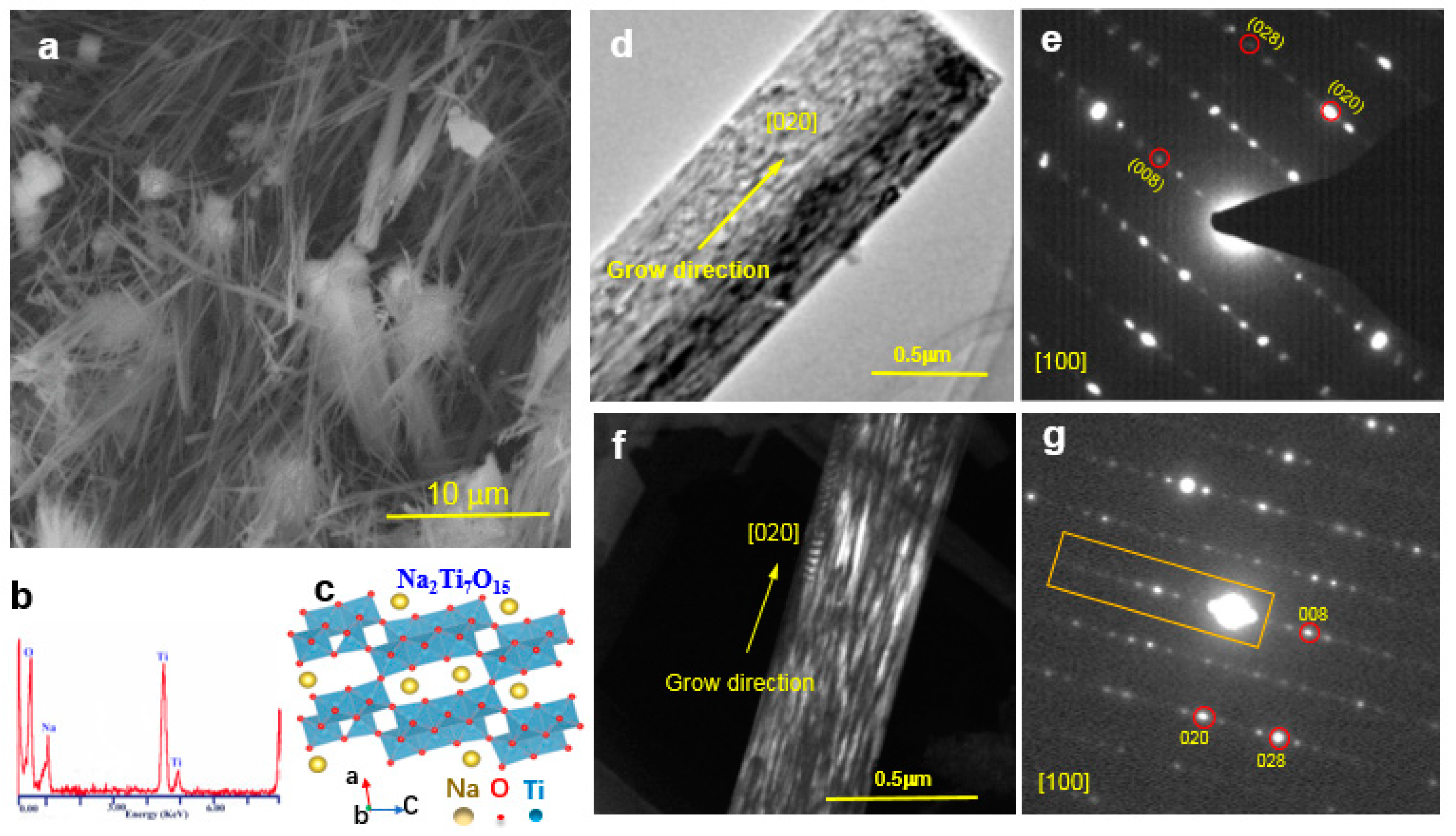This image is a composite of seven grayscale images arranged in a grid and labeled A through G. Each image is square-shaped and includes a yellow scale line for measurement. Image A features a magnified view of intricate, hair-like fiber structures, densely intertwined, with some parts more highlighted than others and a scale indicating 10 nanometers at the bottom right. Image B presents a line chart depicting energy on the x-axis with notable peaks highlighted in red and corresponding chemical elements in blue, including oxygen (O), sodium (Na), and titanium (Ti). Highlighted peaks represent the presence of these elements. Image C shows a detailed 3D chemical composition model labeled Na2Ti7O15. 

Image D illustrates a diagram of material growth direction, annotated with a 0.5-nanometer scale. Image E displays several bright white dots, with some circled in red and numbered 028, 020, and 008 in yellow, suggesting specific points of interest. Image F, similar to image D, shows the directional growth but from a different angle, also with a 0.5-nanometer scale. Finally, image G, akin to image E, includes bright white dots with three circled in red and numbered 028, 020, and 08 in yellow, and a label indicating 100 at the bottom left, taken from yet another angle. The comprehensive details from these images suggest they are high-resolution scientific analyses, likely microscopic in nature.